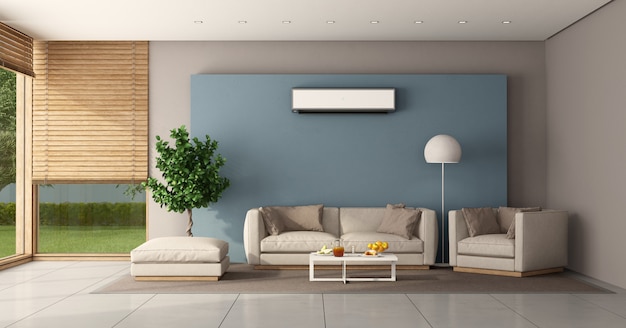The image captures a modern living room in daylight, characterized by large square white tiles with gray grout at the bottom. Centrally, you'll find a beige love seat accompanied by matching cushioned armchair, both adorned with tan throw pillows. An ottoman sits to the left of the love seat, next to a small tree with a twisted trunk and green leaves. In front of the seating area lies a small white coffee table. The background features a grayish-blue rectangular wall panel with a horizontal white rectangle, possibly a light fixture, mounted above. To the right of the armchair, there’s a white lamp. The room boasts a mix of beige walls and a light tan ceiling. On the left side, large windows with natural wood blinds are partially open, revealing green grass and plants outside. The overall ambiance is airy and modern, enriched by the ample natural light streaming through the windows.